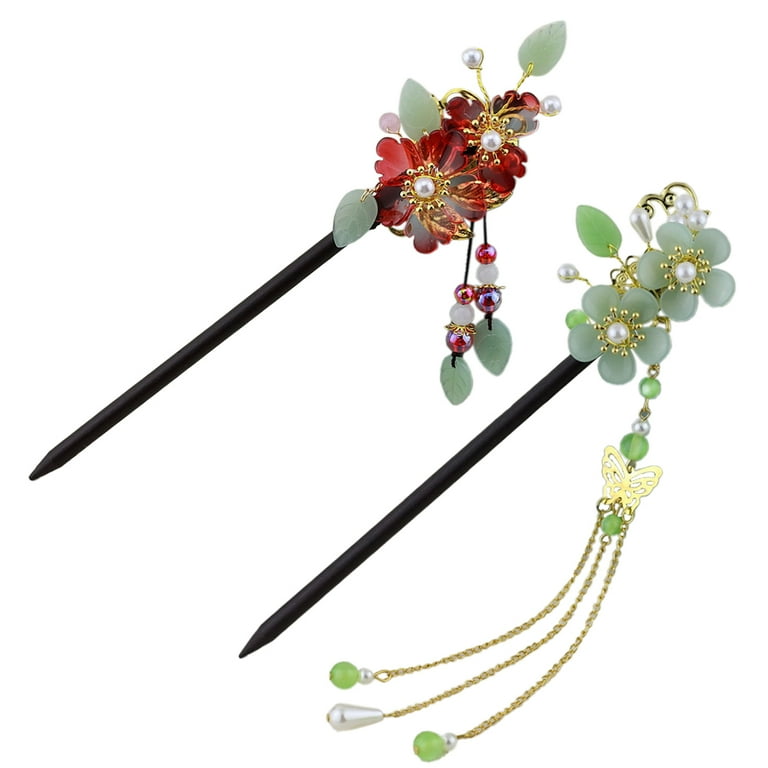The image features two traditional Japanese hairpins, both black and displayed diagonally parallel to each other, with the tops pointing towards the upper right corner and the bottoms towards the lower left. Each hairpin is adorned with intricate floral ornaments at one end. 

The first hairpin showcases two vibrant red flowers with white and gold centers. Delicate light green leaves, possibly made of jade or a similar material, extend from the flowers. Two sets of beads dangle from the floral arrangement, consisting of white, purple, and pink beads, complemented by small white leaves at their ends.

The second hairpin features two off-white flowers with gold centers and a pearl embedded within each bloom. From this ornament, a gold butterfly is attached, supporting three dangling gold chains. Each chain ends with a combination of small white pearls and green beads, with one chain featuring a larger white pearl.

Both hairpins combine elements of traditional Japanese aesthetics and delicate craftsmanship, making them ideal for decorative and functional use in hairstyling.